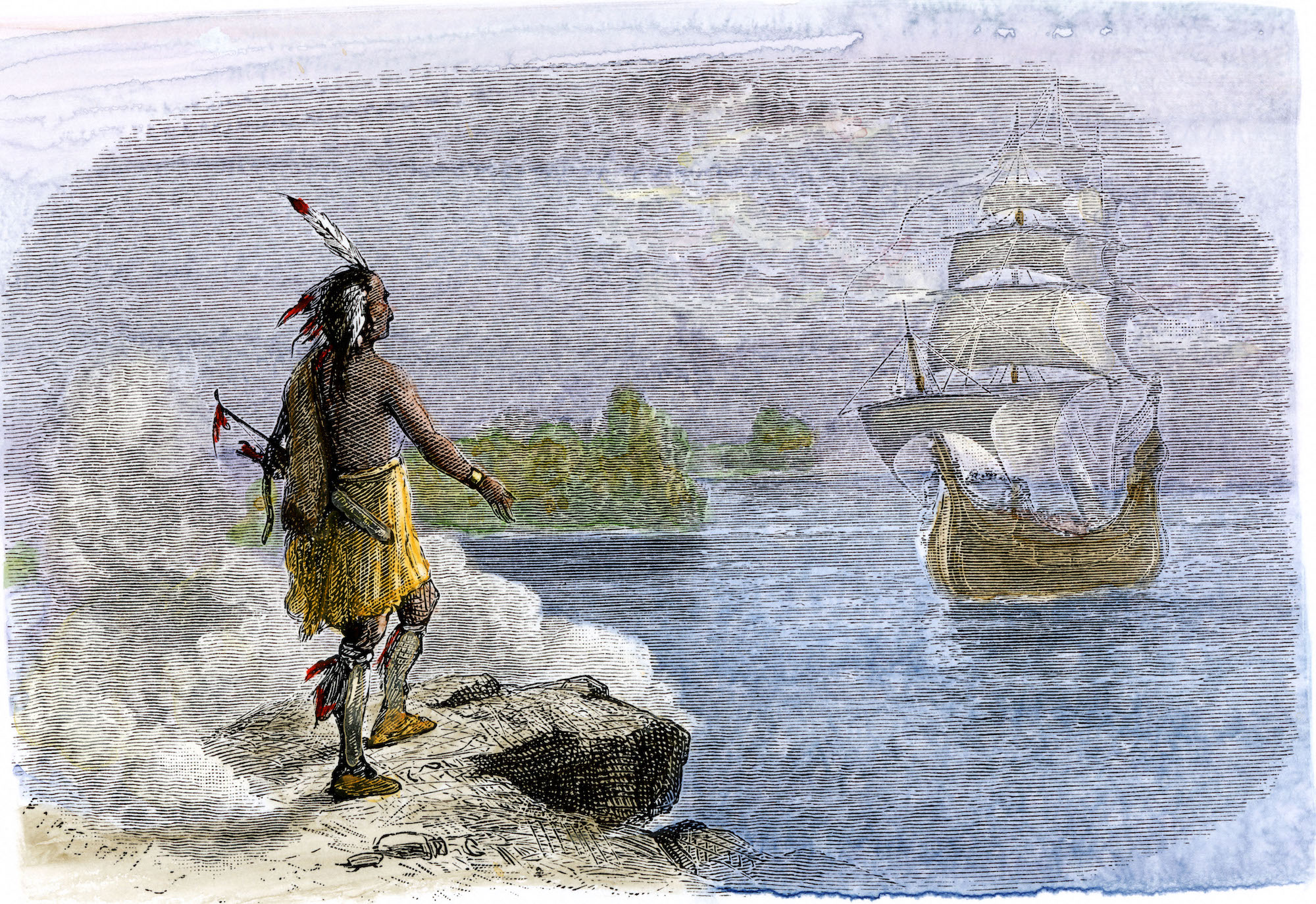The image is a detailed painting that illustrates a 17th-century Native American man standing on a brown rocky outcropping, gazing out over a calm body of water. The man's long black hair, adorned with white feathers tipped in red, flows down his back. He has a dark red complexion and is dressed in a yellowish-brown skirt that extends just above his knees, complemented by high, fabric socks and yellow-brown leather shoes or sandals. A gold bracelet adorns one wrist, and he appears to have a bow and arrow slung over his left arm.

The man is situated amidst some white clouds or fog that partially obscure his legs, adding a mystic aura to the scene. He stands facing a large wooden sailing ship with white sails and rope, approaching from the water. The ship, reminiscent of a pirate or cargo vessel, cuts through the bluish tones of the body of water that show subtle variations of light and dark blue.

In the distance, islands with tree lines populate the horizon, their green foliage faintly visible. The cloudy, grayish sky above suggests daylight, despite its overcast appearance. Surrounding the entire painting is a blue border, adding a finishing touch to this evocative and historical illustration.